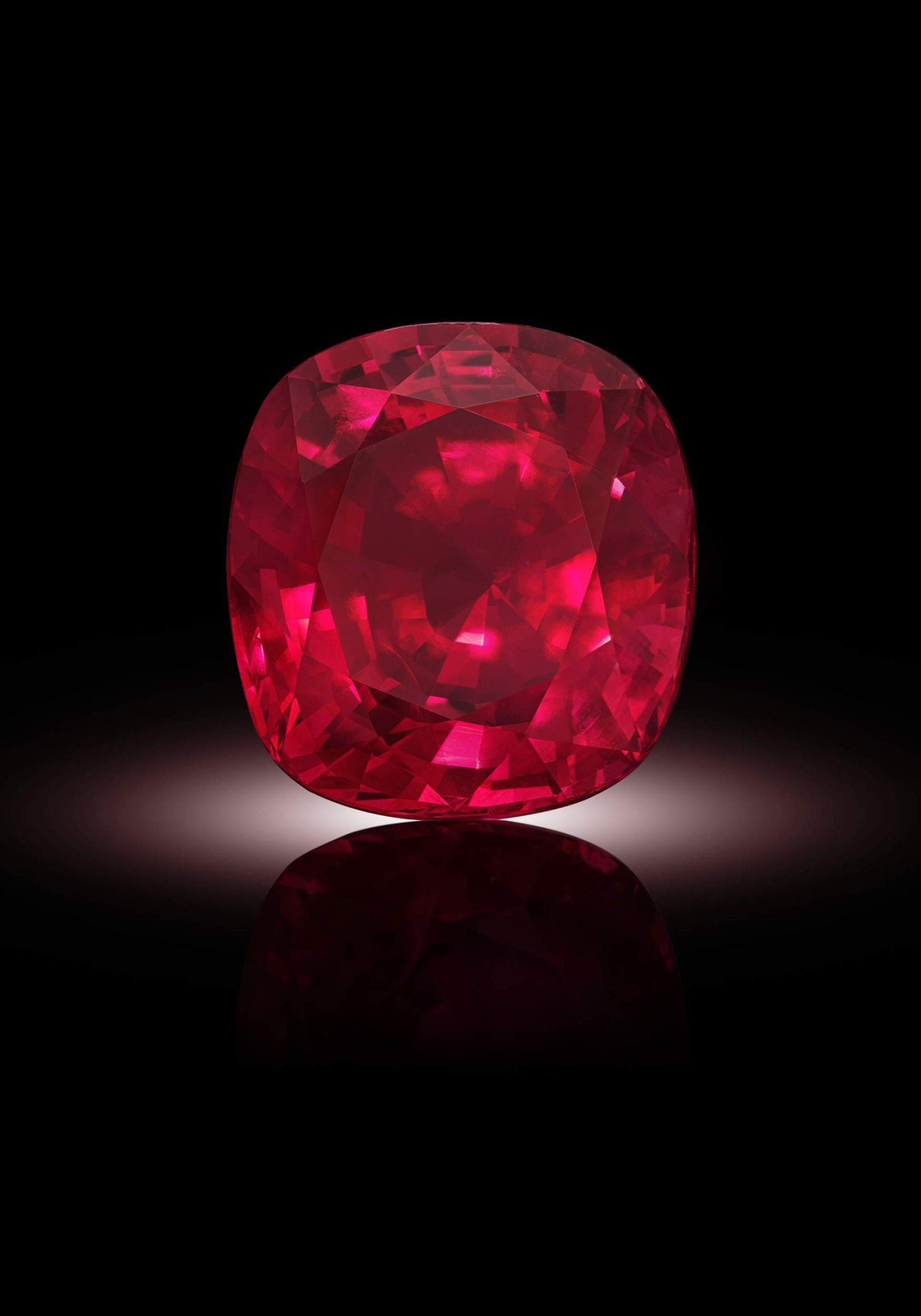The image depicts a magnificent, large ruby standing upright against a stark black background. Positioned on a white, semi-circular platform that serves as the focal point, this deep burgundy gemstone captivates with its multitude of facets. The scene is dramatically lit by a single, concentrated spotlight from below, which not only illuminates the ruby, revealing a dazzling array of red hues and sparkling reflections, but also casts its vivid reflection onto the bright surface beneath it. The reflection mirrors the ruby's size and shape, creating a captivating visual symmetry. Despite the dark background, the intricate details and rich colors of the ruby are beautifully highlighted, making the gem appear almost luminous.